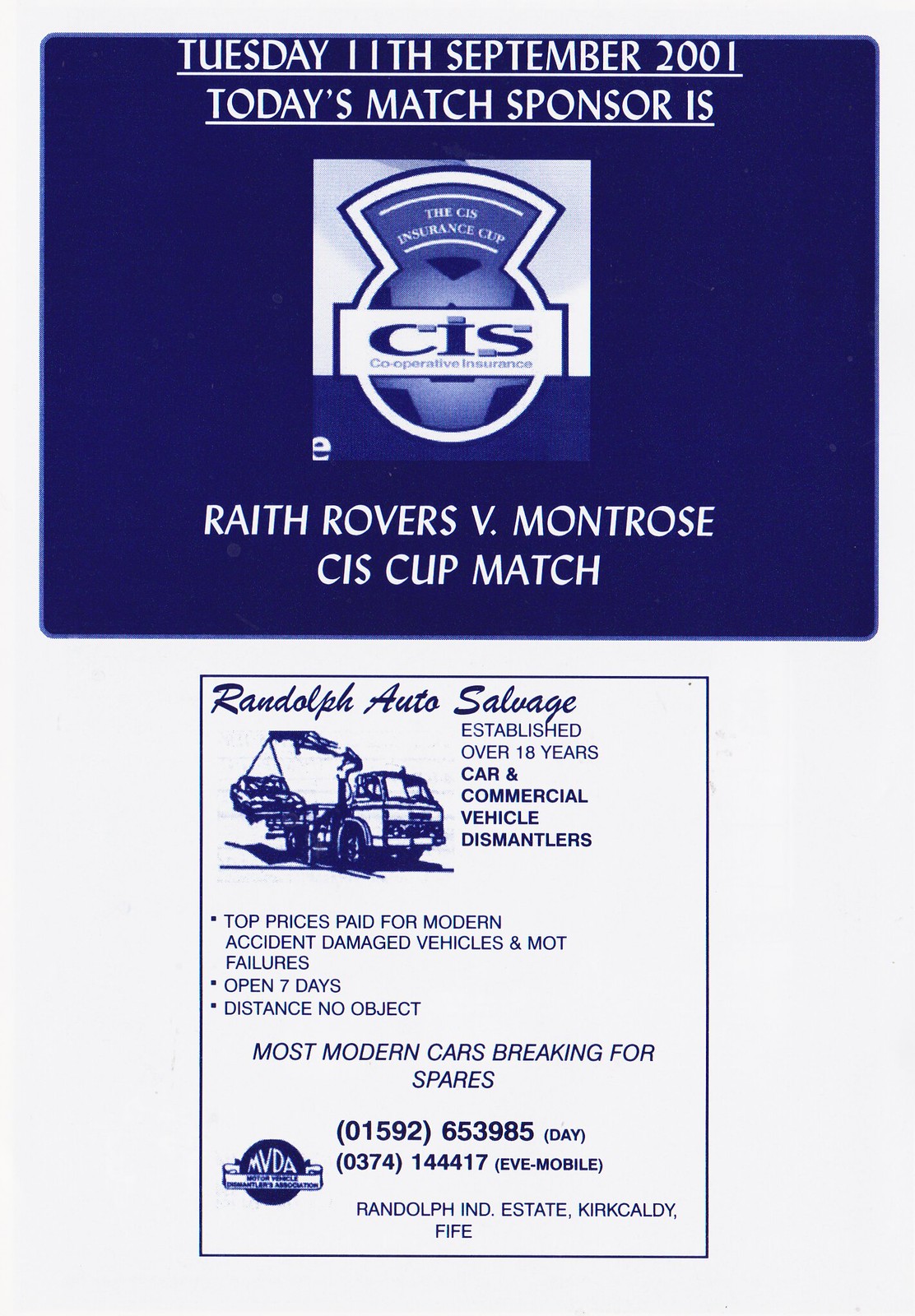This vintage advertisement from the UK is notable for its date, Tuesday, 11th September 2001, the day of the 9/11 terrorist attacks in the United States. At the top of the ad, a dark blue rectangle features white capital letters highlighting the date and the match details: "Today's Match Sponsor is" followed by "CTS," displayed alongside their blue and white logo. Below this, it announces the football match, "Raith Rovers vs. Montrose CIS Cup Match."

Beneath this announcement, there's a prominent advertisement for "Randolph Auto Salvage" written in blue cursive letters. The ad contains a sketched industrial truck and several details in all-blue print. It reads "Established Over 18 Years, Car and Commercial Vehicle Dismantlers," followed by a promise of "Top Prices Paid for Modern Accident Damaged Vehicles and MOT Failures." Additional services and terms include "Open Seven Days," "Distance No Object," and "Most Modern Cars Breaking for Spares." The ad also lists several contact numbers, including a daytime contact and a mobile number, along with an address. This vivid snapshot serves as a poignant reminder of a football match held on a date that would become historically significant.